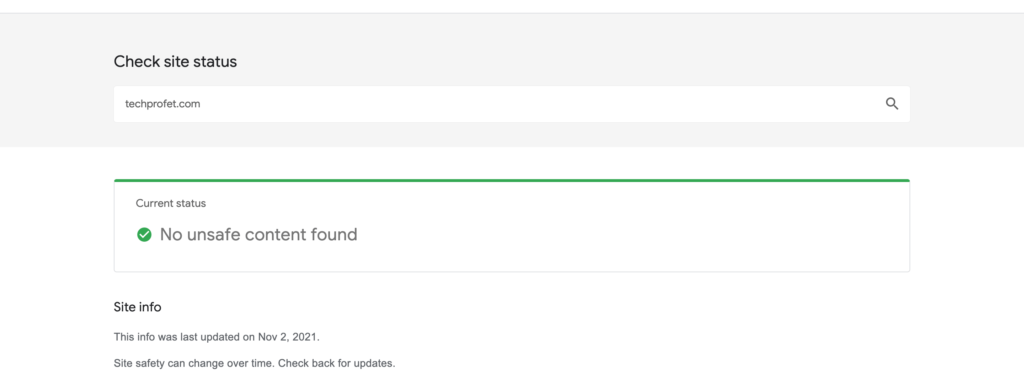The image depicts a webpage designed to check the status of a website. At the top of the page, within a gray header, there is a lighter section containing a search bar that reads "TechProfit.com." Above this, the text "Check Site Status" is prominently displayed. 

Below the header, a green line tops a white information box labeled "Current Status." Inside this box, a green circle with a check mark is prominently featured alongside the reassuring message "No Unsafe Content Found." 

Further down, the section titled "Site Info" provides additional details, stating that the information was last updated on November 2, 2021, and advises users that site safety can change over time, suggesting they should check back periodically for updates.